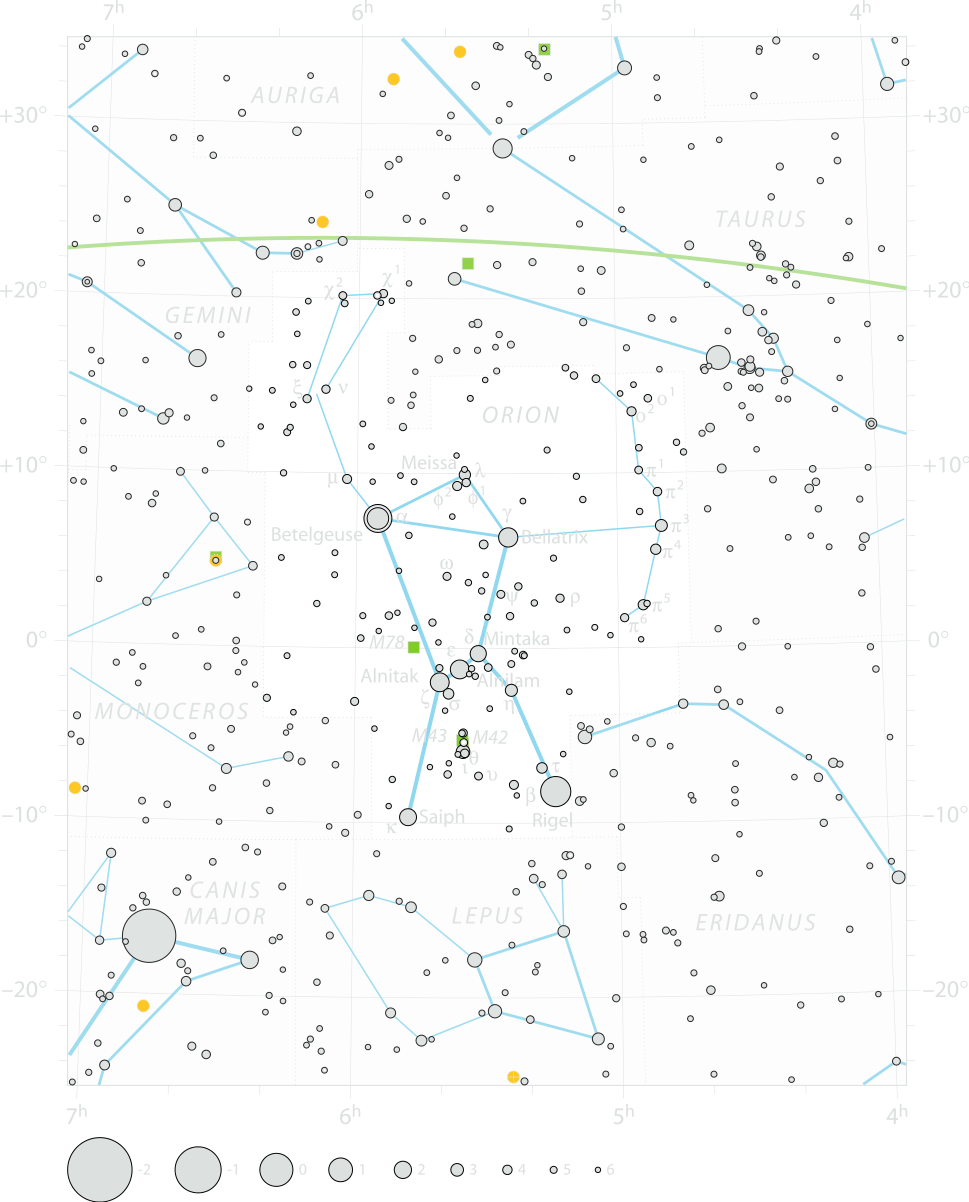The image displays an intricate constellation diagram set against a white background. Blue lines connect various stars to form recognizable shapes and figures. In the top left corner, a triangular formation of blue circles represents the constellation Auriga, labeled in gray text. Moving to the top right, more blue lines outline the constellation Taurus, also labeled in gray. Prominently in the center, the well-known constellation Orion is depicted. Smaller constellations are scattered throughout, including Canis Major in the bottom left corner. A key at the bottom, with a gradient of bubble-like circles ranging in size, explains the significance of each circle. Names like M78, Mintaka, Alnitak, and Monoceros feature within the map. The diagram includes lines to denote positional coordinates, enhancing the navigational aspect of the star map.